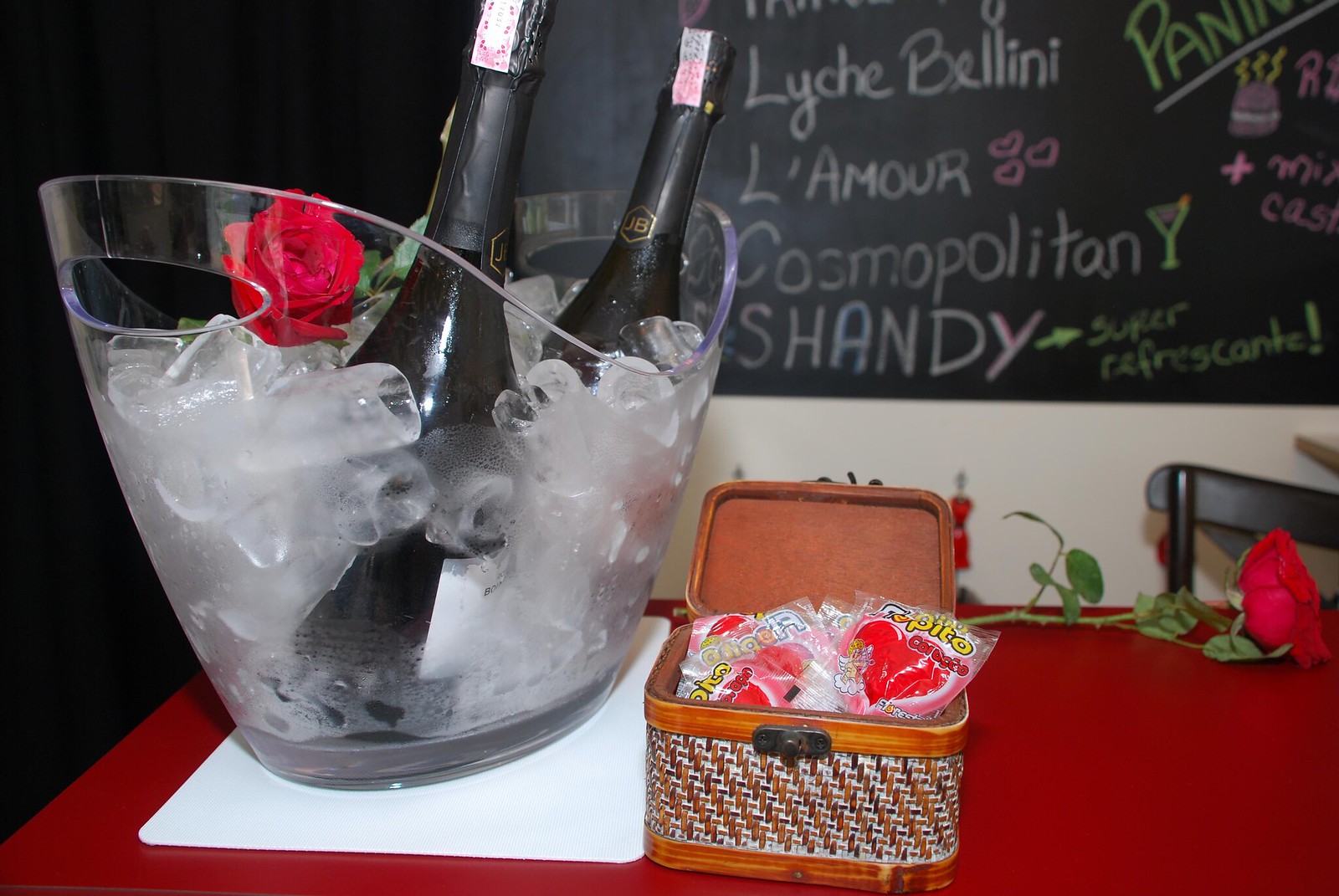The photograph captures a festive event setting featuring a prominently displayed ice bucket with two bottles of champagne, partially submerged and marked with a logo resembling "JB" inside a hexagon. A single rose is nestled among the ice. Adjacent to the ice bucket, a traditional bamboo box with its lid open reveals small red packages adorned with hearts and a cupid motif. The table, covered with a vibrant red tablecloth, also supports another delicate rose. The background is dominated by a chalkboard wall listing various cocktail options like Lychee Blini, L'Amour, Cosmopolitan, and Chamois, described as "super refreshing," embellished with colorful chalk drawings of drink glasses, hearts, and love signs. Black wooden chairs are positioned nearby, completing the celebratory ambiance.